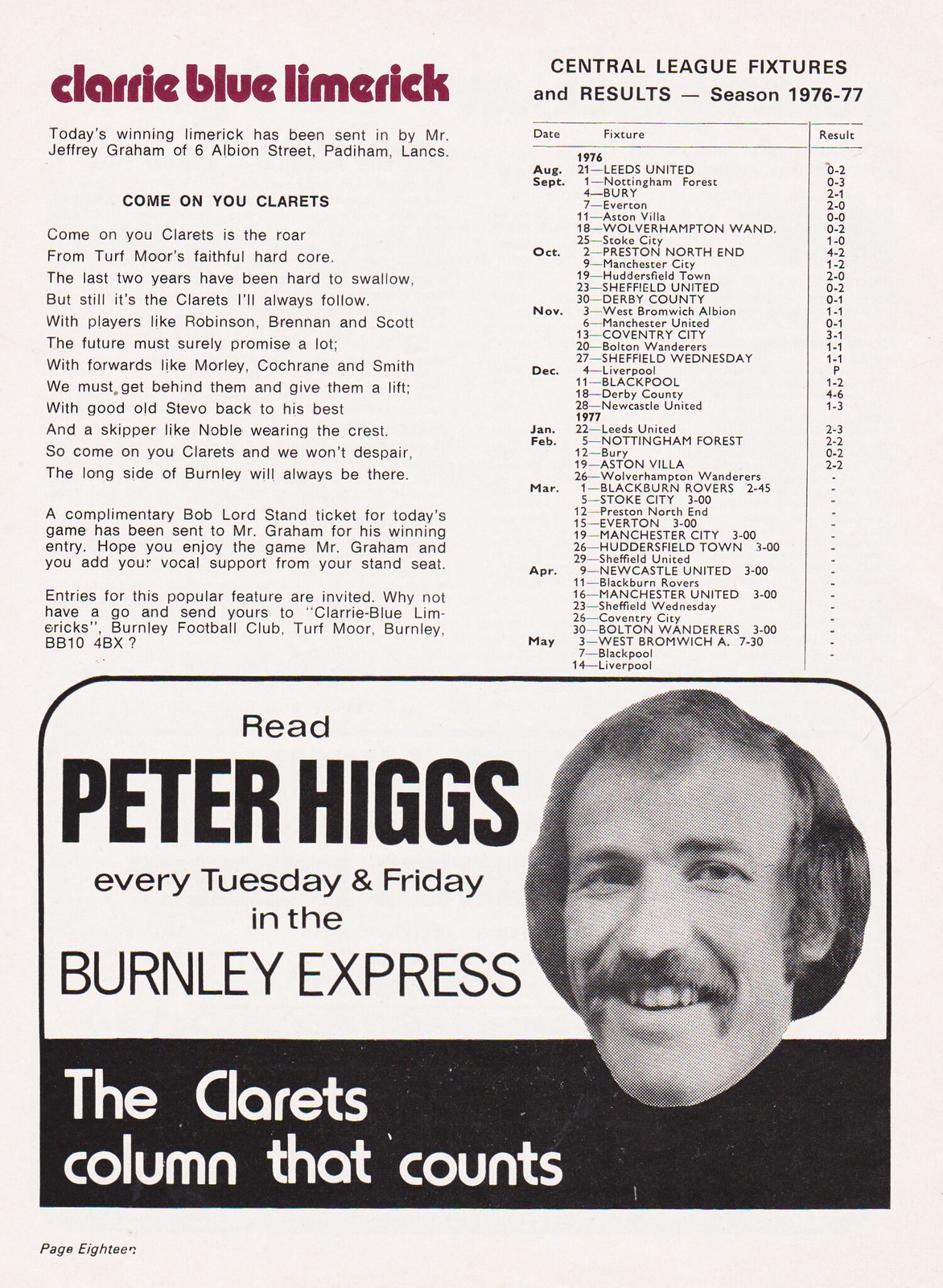This image displays page 18 of an old soccer program, likely from a Burnley football magazine, featuring content from the 1976-1977 season. The background holds a faded pinkish tint and the top left corner includes the heading "Clary Blue Limerick" written in a stylized red or maroon lowercase font. Beneath this title, it reads, "Today's winning limerick has been sent in by Jeffrey Graham of 6 Albion Street, Padiham, Lancs." The limerick, titled "Come On You Clarets," celebrates Burnley FC’s team spirit and loyal supporters. Details of the players and a shout-out to their commitment are highlighted in the poem. For his winning entry, Mr. Graham is awarded a complimentary Bob Lord Stand ticket for the game.

On the right, the page lists the Central League Fixtures and Results from August 1976 to May 1977. The results up to February are provided, showing scores from various matches, such as Leeds United's 2-3 on January 22 and Nottingham Forest's 2-2 on February 5, while matches from late February to May are listed without results, indicating they had yet to be played at the time of publication.

The lower section of the page features an advertisement for a columnist named Peter Higgs, promoting his columns in the "Burnley Express" which appear every Tuesday and Friday. A headshot of Peter Higgs depicts him as a mustached man with shaggy hair and a welcoming smile. Below his image, a black bar with white text states "The Clarets Column that counts," likely reaffirming his dedication to covering Burnley FC.

Overall, this page radiates the passionate essence of Burnley FC supporters, offering an engaging mix of creative writing, match updates, and local journalism.